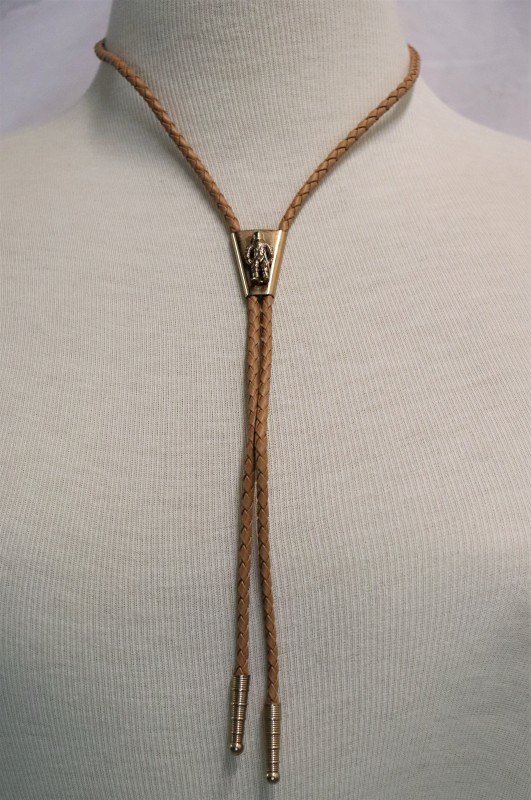This indoor, color close-up photograph captures a detailed view of a product modeled on a mannequin, which is depicted from the neck down dressed in a white, vertically-textured woven fabric. Centered around the mannequin's neck is a braided brown bolo tie, resembling a shoelace, with a distinct gold trapezoidal clasp positioned at the neckline. The metal clasp, exhibiting a 3D-like embossed image of a person, holds the two strands of the bolo tie together. The bolo tie ends with metal finials hanging mid-chest, adding a subtle yet striking contrast to the minimalist white fabric. The entire setup, devoid of any head or arms in view, highlights the new and intricate craftsmanship of the necklace against a plain white background.